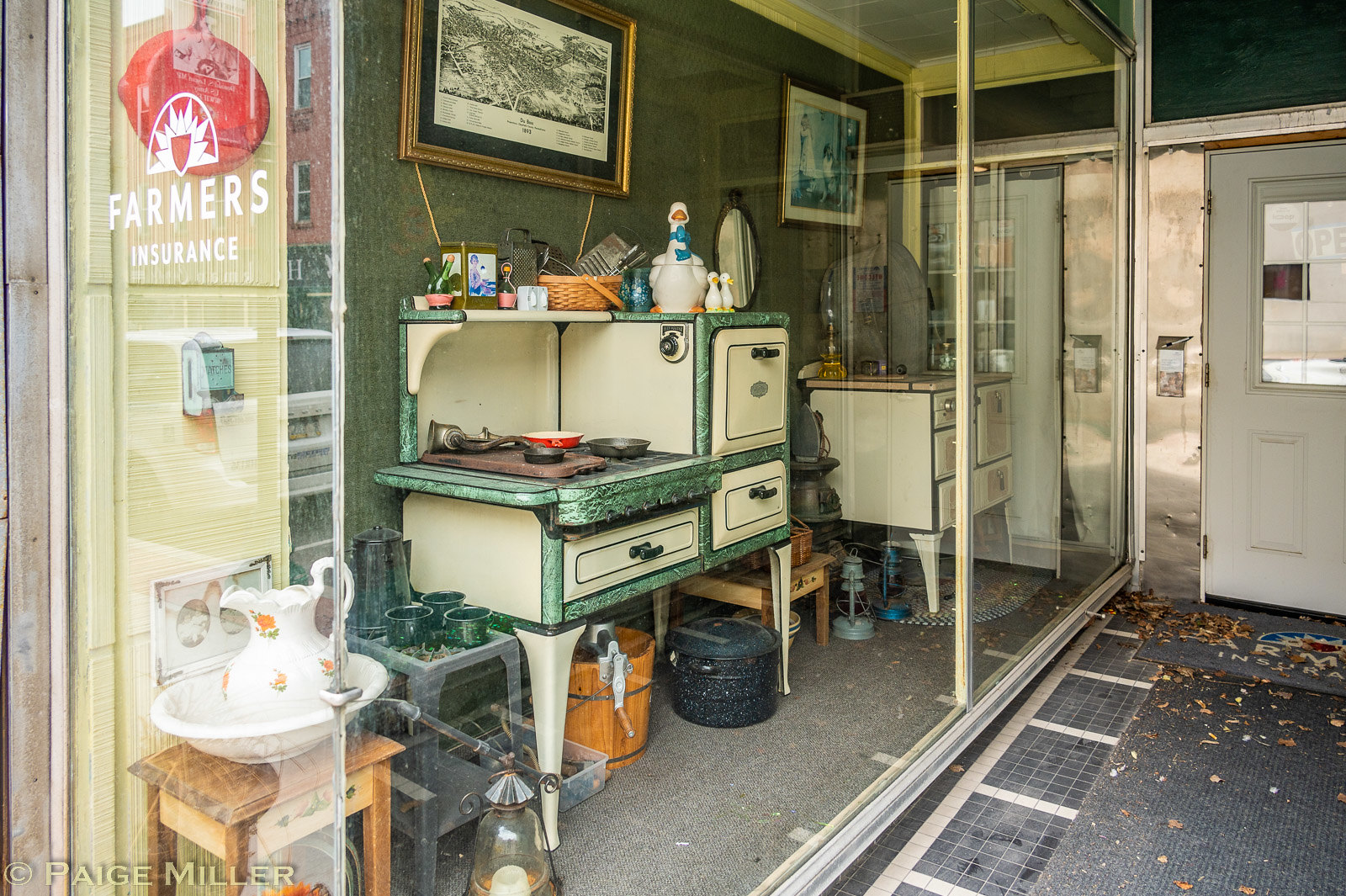The image captures a showroom display next to a store, entirely enclosed in glass with the text "Farmer's Insurance" prominently displayed on the front window. Inside, there is an antique kitchen setup featuring a vintage stove in white and turquoise, possibly with an attached oven. Below the stove, there are two buckets: a metal black one and a wooden brown one. Adjacent to the stove, on the right, is a white dresser or cabinet with pullout drawers. The scene also contains a white teapot with floral designs on a stand near the front of the enclosure. Above the stove and the dresser area, framed pictures adorn the walls. In the background, to the right, a modern white door with a glass window provides an entrance to view the display. The entire setting suggests a museum-like exhibit of an old-style kitchen, meticulously arranged and visible through the glass panes.